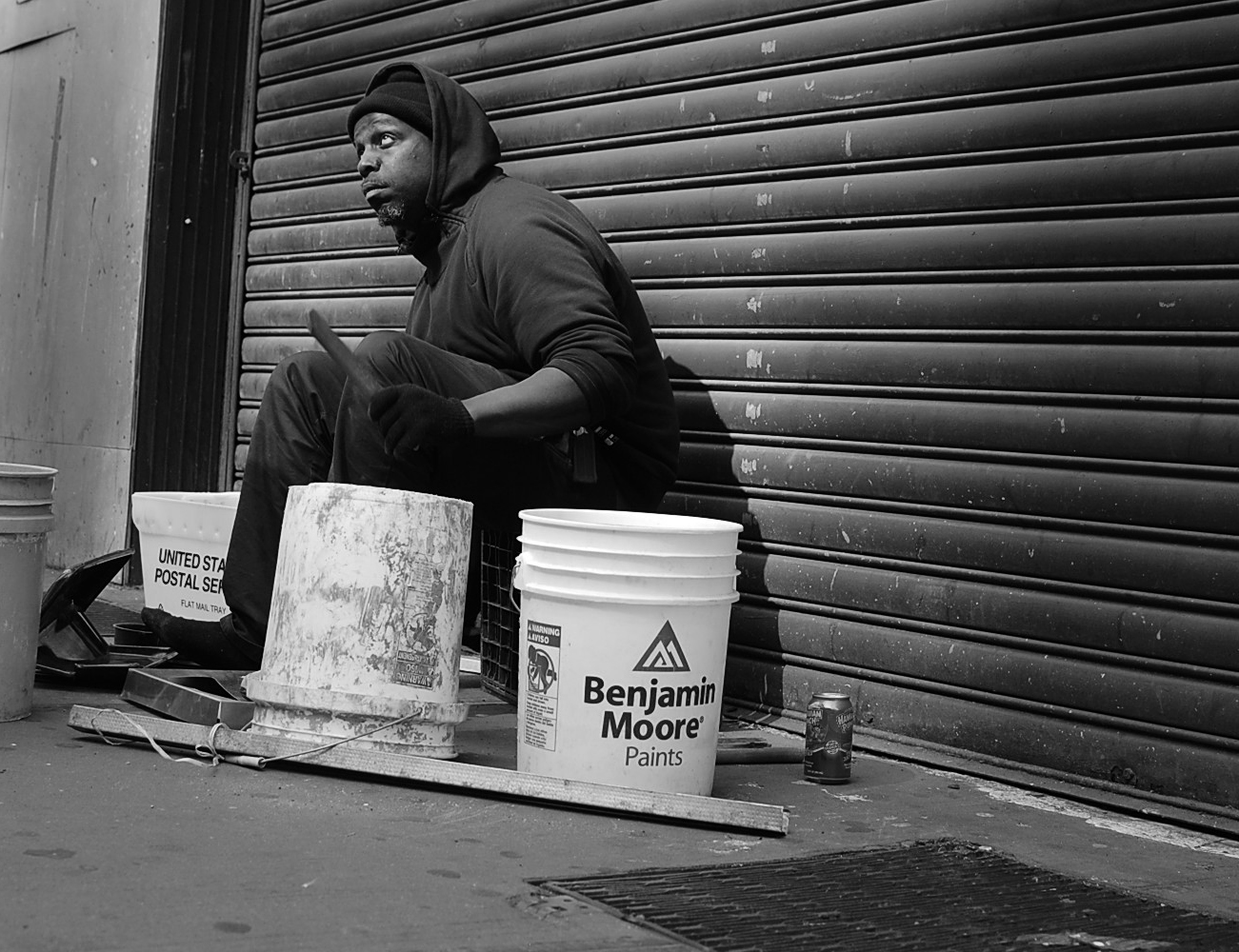This black-and-white photograph captures an African-American man seated on an urban sidewalk in front of a closed metal gate. He is perched on a black box, or perhaps a plastic milk crate, surrounded by various items that paint a vivid picture of his surroundings. To his left are two white five-gallon paint buckets, one upright and labeled "Benjamin Moore," and the other overturned. Beside these buckets is a can of soda, and nearby stands a white plastic U.S. Postal Service bin. In front of the man sits another bucket, and there is a grate integrated into the sidewalk. A wooden plank lies on the ground, adding to the array of objects. The man, who sports a mustache and goatee, is dressed warmly in black attire, including black pants, a black hoodie with the hood up, and a black cap underneath. He also wears gloves and appears to be gazing up at the sky. The scene suggests a bustling urban environment, with the possibility that the man might be using the buckets as makeshift drums, perhaps to perform for passersby.